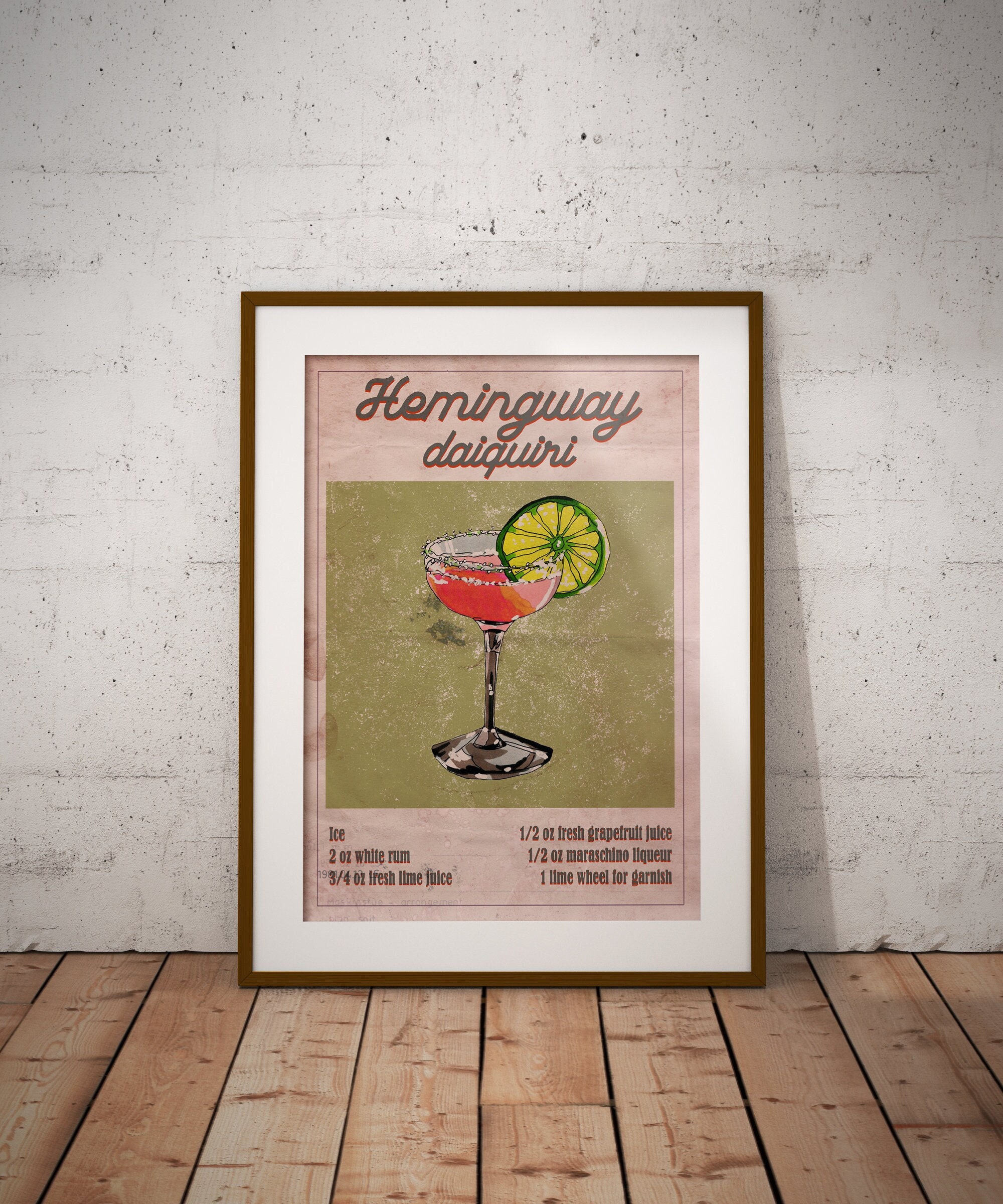This image captures a square color photograph of a framed print resting against a white, distressed wall. The hardwood floor, composed of medium-toned wooden planks, subtly complements the setting. The main focal point is a thin brown wooden frame, inside which a white matting surrounds the print titled "Hemingway Daiquiri" inscribed in elegant cursive. Below the title, an illustrated daiquiri is depicted in a champagne-like rounded stemmed glass, holding a pink liquid with a large lime or lemon wedge garnishing the rim. The artwork further details the cocktail recipe, listing ingredients: ice, 2 ounces of white rum, ¾ ounce of fresh lime juice, ½ ounce of fresh grapefruit juice, ½ ounce maraschino liqueur, and 1 lime wheel for garnish. The framed print casts a slight shadow on the right, enhancing the depth and texture of the scene.